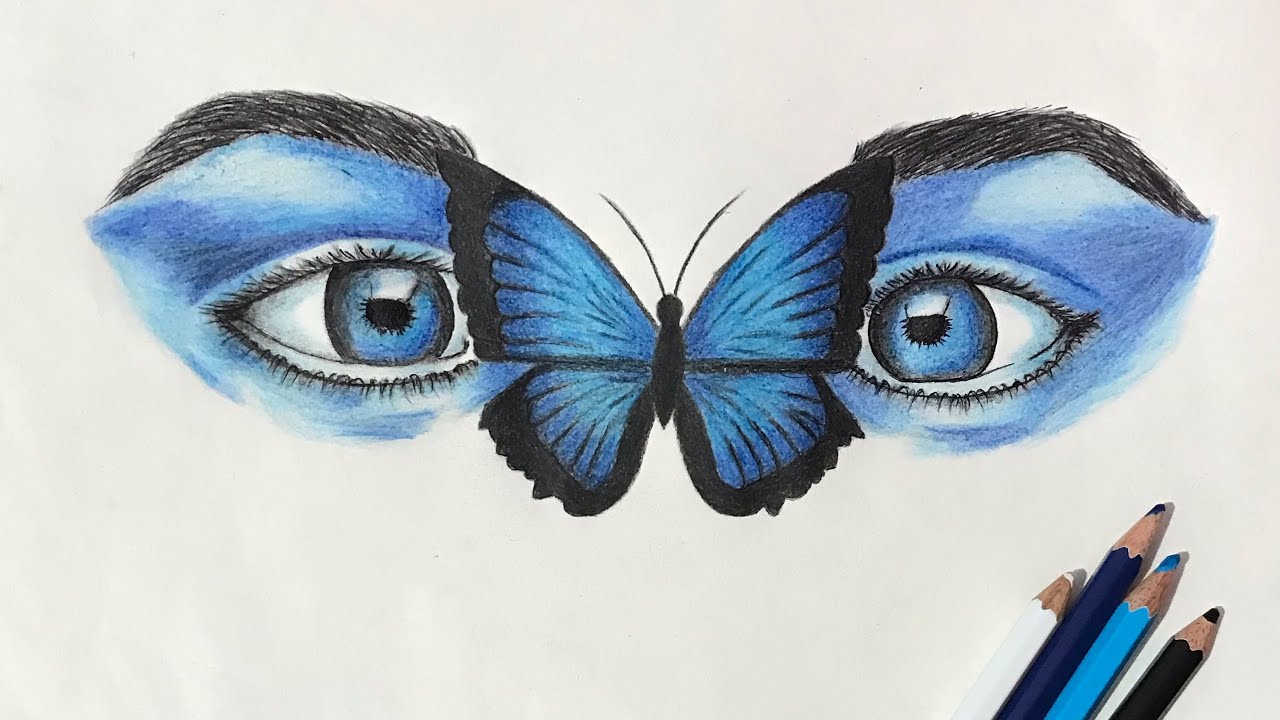The image is a colored pencil drawing featuring a close-up of two eyes on a cream-colored background. Each eye boasts striking blue irises that match the blue ink shading the eyelids and surrounding area. The pupils are black, and the eyes are framed by prominent black eyelashes and dark eyebrows. Between the eyes rests a detailed blue butterfly with black borders on its wings and a black body, complete with visible antennas. In the lower right corner of the image, three colored pencils—white, navy, turquoise, and black—are arranged diagonally side by side, their tips visibly pointing towards the center. The background remains predominantly light to enhance the vivid blue and black elements of the drawing.